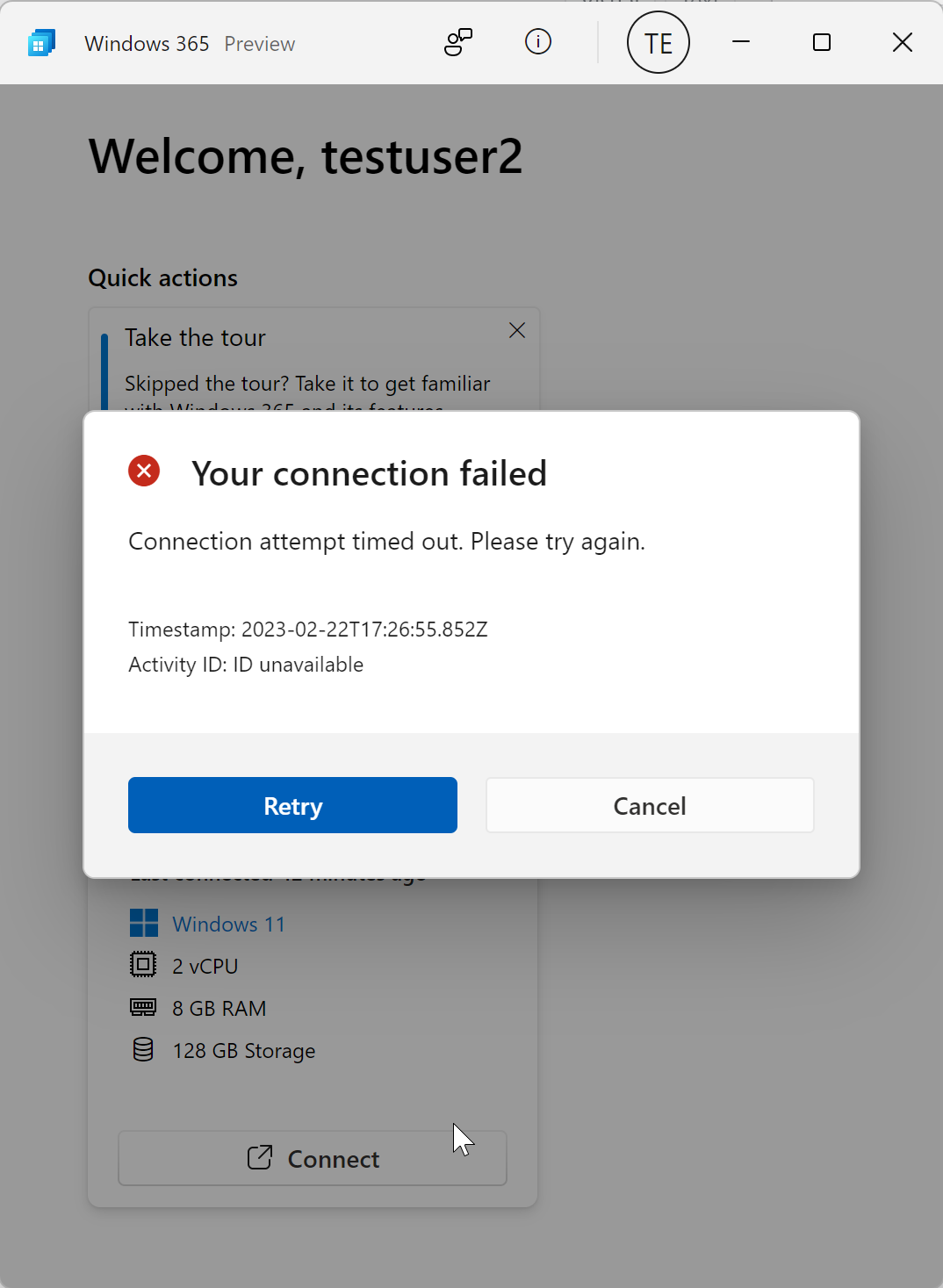The image shows a Windows 365 preview page overlayed with a semi-transparent gray filter. On the underlying page, it welcomes the user identified as "test user 2" and offers quick actions such as "Take Tour", "Skip the Tour", and "Get Familiar".

Over this, a white pop-up message appears, indicating a connection failure. The pop-up features a red circle with a white 'X' icon and a message that reads: "Your connection failed. Connection attempt timed out. Please try again. Timestamp: 2023-02-22T17:26:15.852Z. Activity ID: ID unavailable". 

The bottom of the pop-up includes a horizontal gray bar housing two buttons: a blue "Retry" button with white text and a white "Cancel" button with black text.

Partially visible beneath the pop-up on the grayed-out background, there are specifications listed for a virtual machine: "Windows 11, 2V CPU, 8GB RAM, 128GB storage". Nearby is a white "Connect" button with black text, over which a white cursor hovers, ready to click.